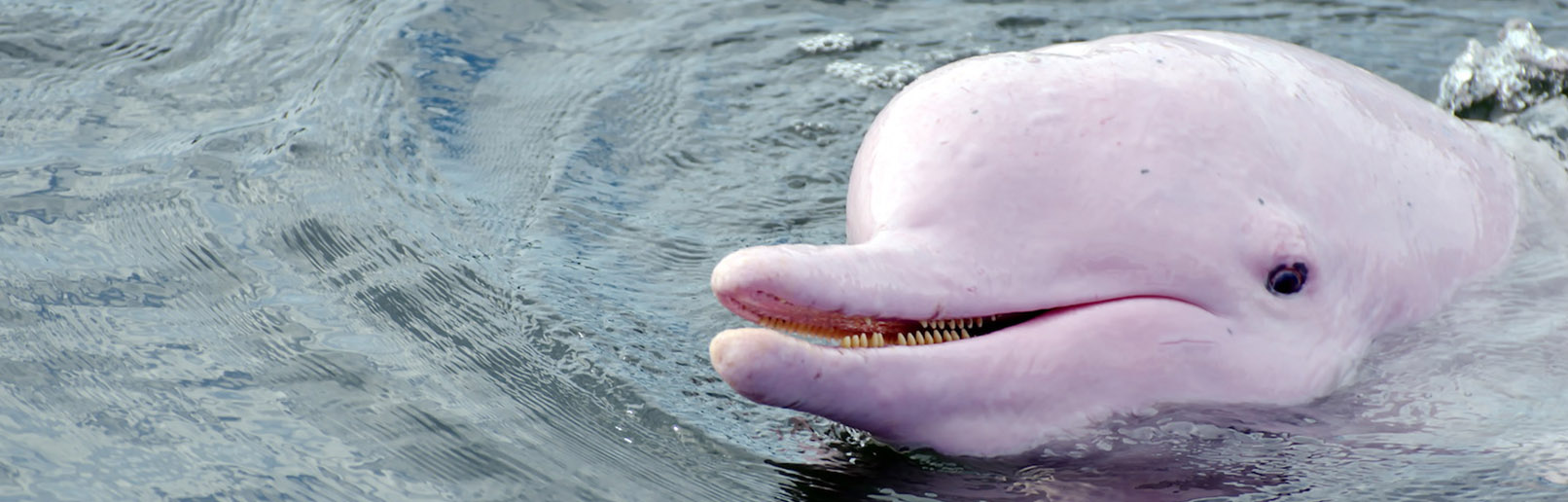In this image, we see a close-up photograph of a pink dolphin, possibly misidentified as a small whale, emerging from a dark blue sea. The image is horizontally cropped and resembles a thin strip, focusing tightly on the dolphin’s head. The dolphin, with its skin resembling that of an uncooked chicken, has its mouth slightly open, exposing its teeth in a goofy, almost smiling expression. The visible eye on the right side of its head looks towards the camera. Bright sunlight illuminates the dolphin's pinkish-colored back, while its head casts a shadow beneath it. The water around the dolphin shows waves and movement, accentuating the action of the creature poking its head out of the sea.